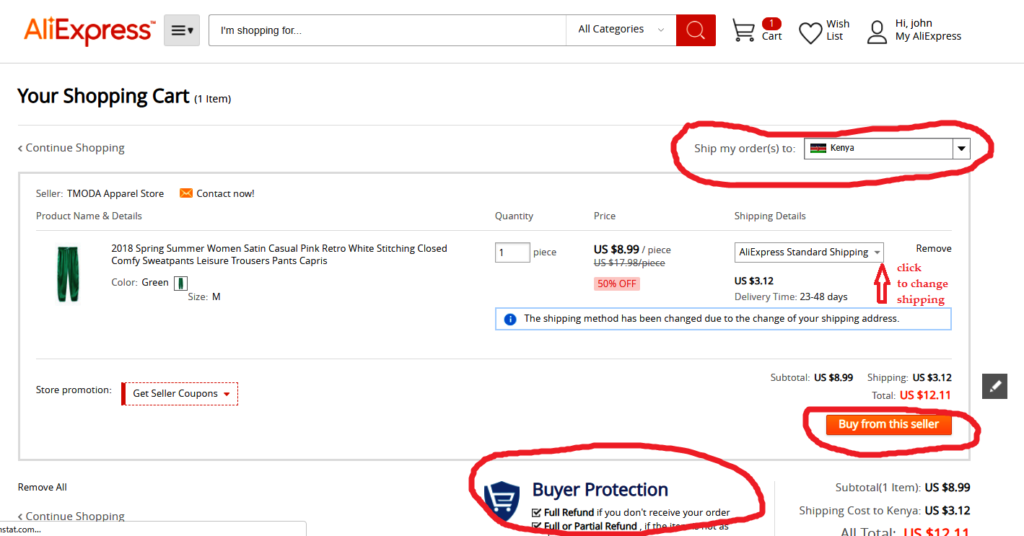**Detailed AliExpress Shopping Cart Screenshot Description**

The screenshot captures a web page from AliExpress, the popular online retail service. At the top of the page, the navigation bar includes an "I'm Shopping For" search box, an "All Categories" drop-down menu, and a cart icon displaying one item. To the right, there are links to the user's wish list and a personalized greeting, "Hi John," leading to the "My AliExpress" section.

In the shopping cart section, a detailed listing of the selected item is displayed. The item is the "2018 Spring Summer Women's Satin Casual Pink Retro White Stitching Closed Comfy Sweatpants, Leisure Trousers, Pants Capris" in green, size medium. The quantity is set to one piece, priced at $8.99 USD after a 50% discount from the original price of $17.98 USD. AliExpress standard shipping is added at a cost of $3.12 USD, with an estimated delivery time ranging from 23 to 48 days.

The subtotal for the selected item is $8.99 USD, with an additional shipping cost of $3.12 USD, leading to a total order amount of $12.11 USD. Notably, the shipping cost to Kenya is confirmed to be $3.12 USD. Several elements on the page are highlighted with red circles, including the option to "Ship my order to Kenya," the "Buy from this seller" button, and information about buyer protection, which guarantees a full refund if the order is not received and a full or partial refund if the item does not match its description.

The overall layout of the page clearly shows that the user is ready for checkout, with all necessary details about the product and shipping costs transparently displayed.